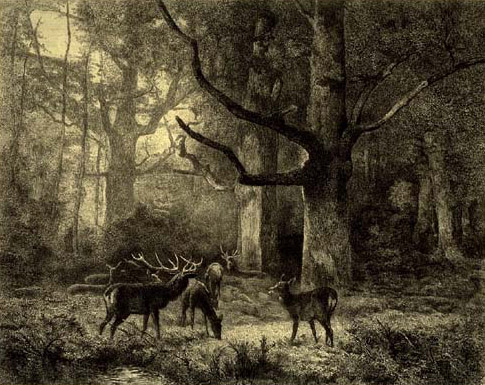This detailed drawing, rendered in monochromatic tones using pencil and possibly colored pencils, depicts a serene forest scene populated by four deer. The central figures include two male deer, identifiable by their antlers, standing alert with heads raised, and two female deer, heads lowered, grazing on the grass. The ground is covered in an abundance of shrubbery and greenery. Dominating the foreground is a large tree, its massive branches extending about ten feet above the deer, showing signs of burns with no leaves, while the background reveals a dense canopy of leafy trees. Light filters through, particularly prominent at the upper-left, indicating a sparser area in the forest that allows sunlight to peek through. In the background, the forest thickens, becoming darker and more densely clustered with trees. This intricate and detailed illustration encapsulates the tranquility and natural splendor of a dense forest environment.